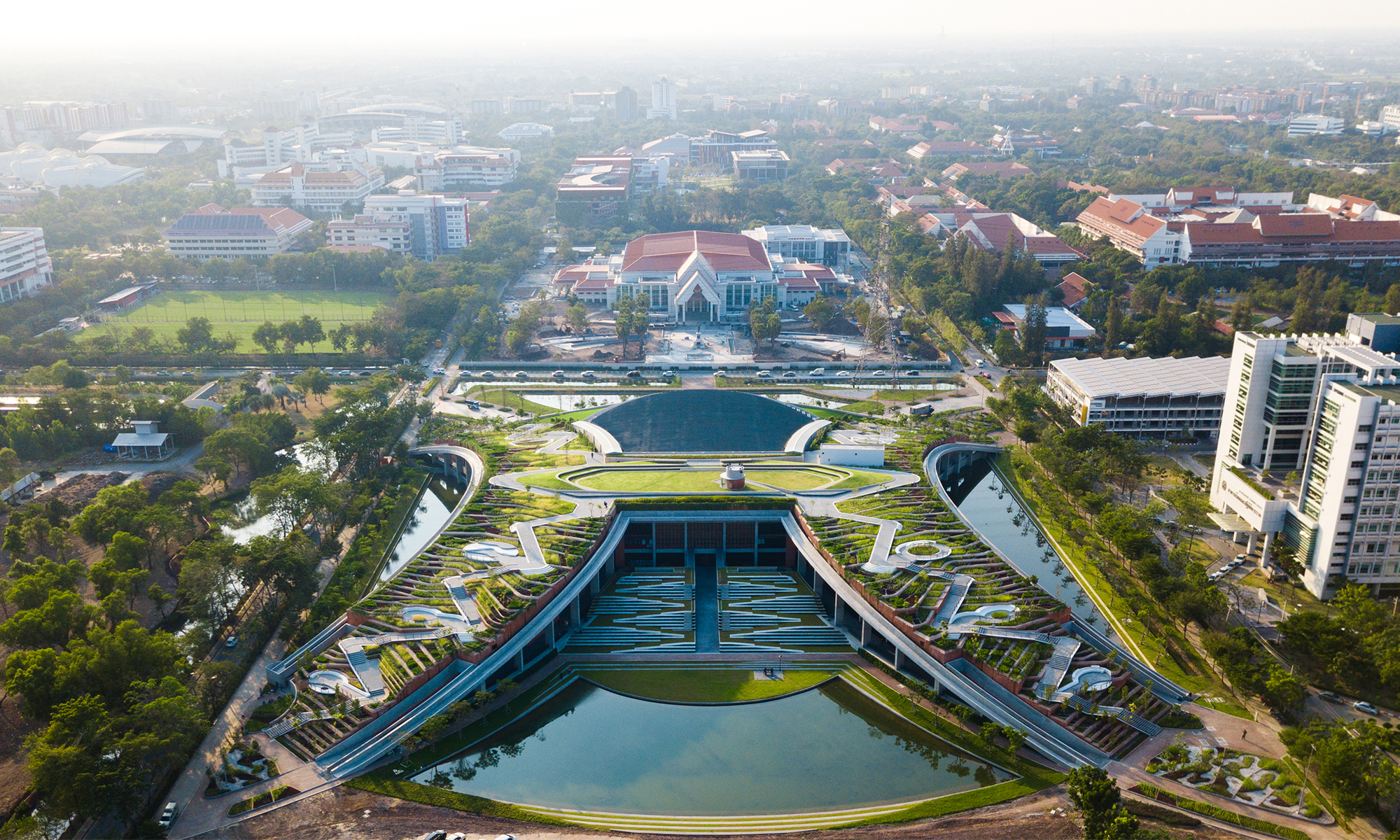The aerial photograph showcases a sprawling urban cityscape dominated by a mix of large and wide buildings, interspersed with green areas. On the left side of the image, there is a generous garden filled with numerous trees and a lush grassy expanse. Centered within the image, a distinctive white building with a red roof, featuring two triangular peaks and an entrance, stands prominent. This building is situated within a patterned square surrounded by bushes and trees, and in front of it lies a substantial structure resembling a stadium. In the foreground, a man-made pond shaped like a wide arc anchors the bottom section of the image. To the right, a tall white building rises, contributing to the city's dense architectural landscape. The city's layout appears meticulously planned, with streets forming a grid pattern and numerous buildings nestled within this orderly arrangement. In the distant background, late into the image, the skyline fades into a whitish hue due to fog or smog, with Little Burry and additional buildings barely discernible.